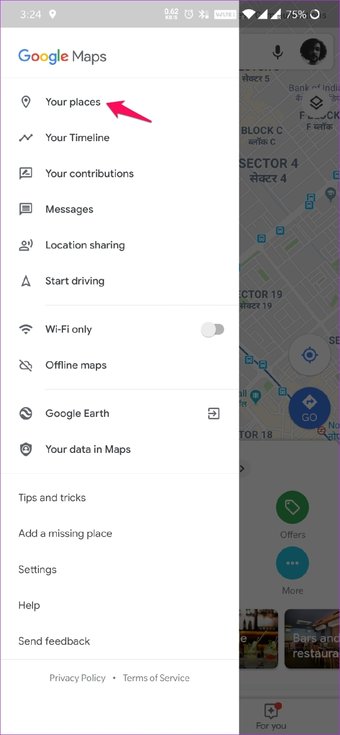This image is a screenshot taken from a mobile phone displaying the Google Maps application. The dimensions are consistent with a smartphone's long rectangular screen, evident by the status bar at the top indicating the time as 3:24 PM, alongside icons for GPS, distance (0.62), an alarm clock, Bluetooth, Wi-Fi, and a battery level at 75%.

The primary focus is on the Google Maps side menu, which occupies most of the left half of the screen. The side menu options listed, each with corresponding icons, include: Your places, Your timeline, Your contributions, Messages, Location sharing, Start driving, Wi-Fi only, Offline maps, Google Earth, and Your data in Maps. An arrow is pointing to the "Your places" option, suggesting that this might be part of a tutorial or guided feature.

On the right side, partially visible behind the menu, is a map displaying a location labeled as "Sector 4, Block C." At the top left of the side menu, there is a highlighted user profile photo. The overall context and highlighted elements imply the user is interacting with or receiving instruction on how to use the "Your places" feature in Google Maps.